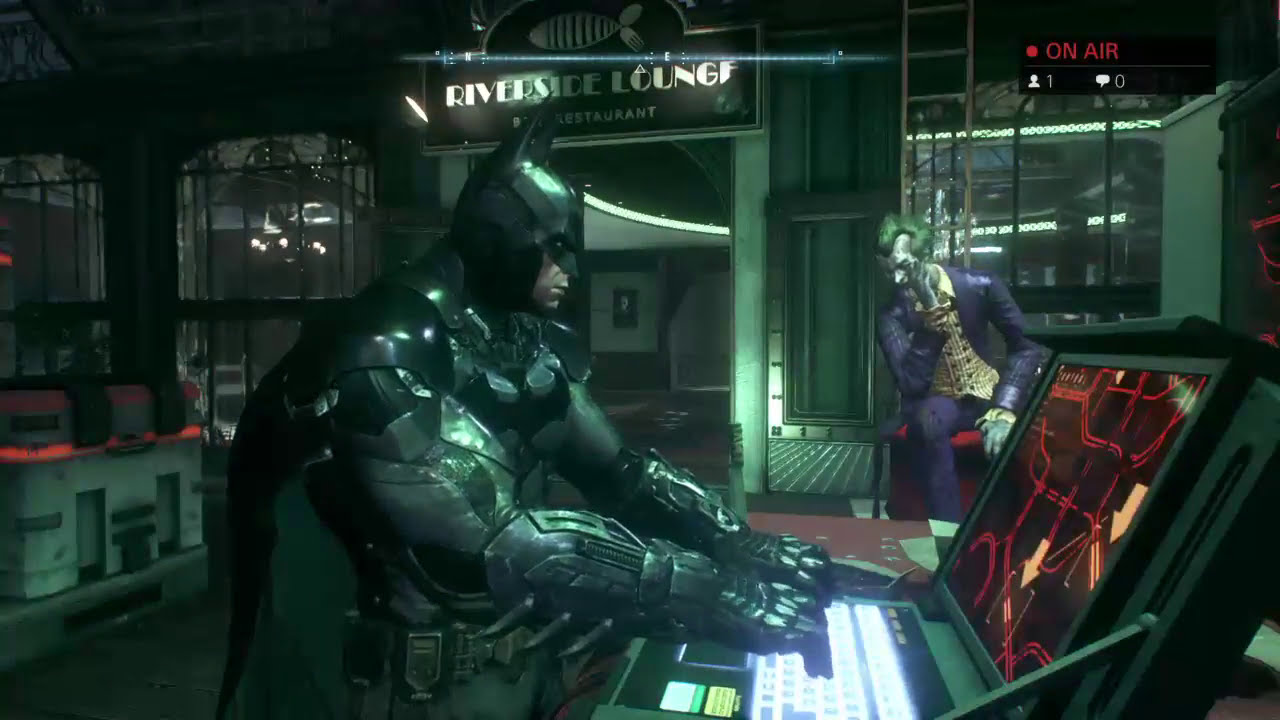This image is a detailed animated screenshot from the game Gotham Knight, capturing an intense scene featuring Batman and the Joker. Batman, dressed in a black cowl with bat ears, a black cape, and a muscular black metal suit, stands slightly left of center, facing right with both hands typing on a backlit, industrial type of keyboard attached to a large monitor. The monitor displays a bird’s eye view of Gotham's city streets with red-lined roads against a black background. The scene appears to be set in the Riverside Lounge, evident from a black sign above a doorway in the background, which has a large white fish and the words "Riverside Lounge" in white letters. The gritty industrial setting is underlined by green metal walls with ornate windows.

To Batman’s left, the Joker with pale skin, green hair, and wearing a purple suit with a yellow shirt, sits on a desk, gesturing towards Batman with one hand in a whisper-like manner. In addition to the main focus, the background reveals further details such as a ladder leading to a second level, a desk area, and the overall nighttime ambiance of a lounge. An "On Air" indicator in the top right corner of the image shows zero chat bubbles, suggesting it’s a streaming or recording scene. The overall environment highlights the tension and complexity of their confrontation.